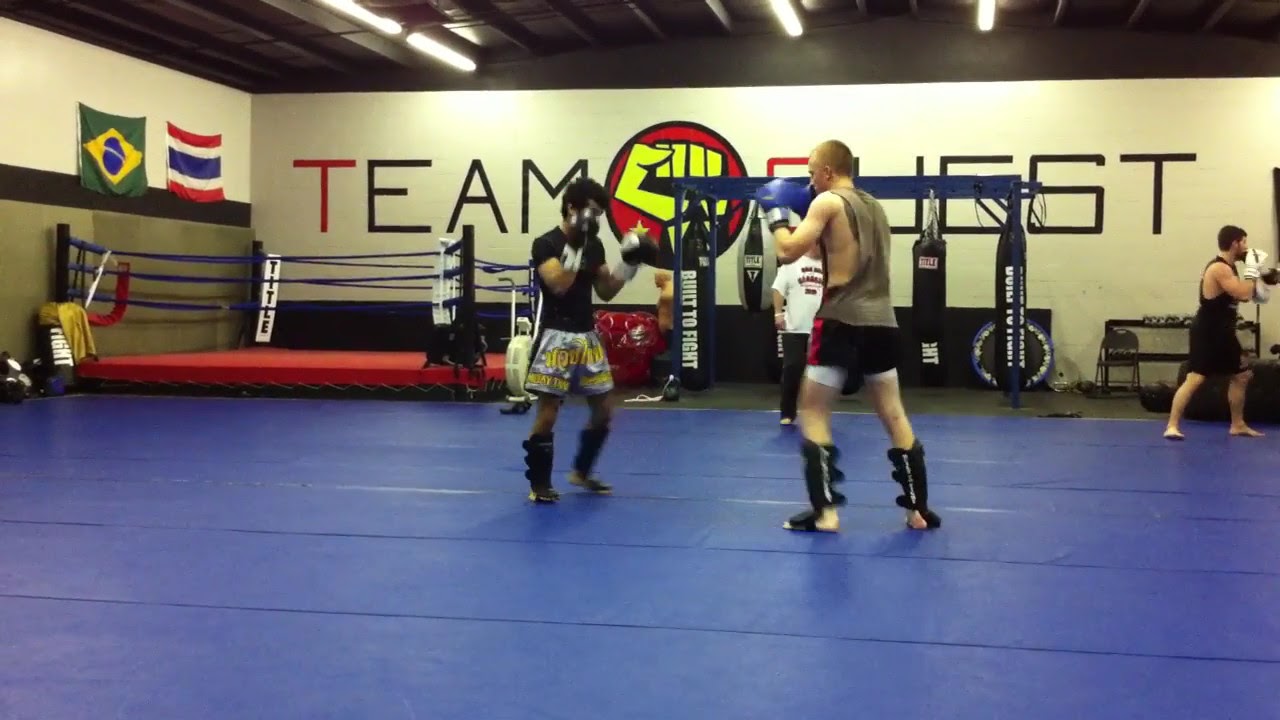The image captures two young men sparring in a mixed martial arts gym, highlighting the rigors of their training. Both are equipped with boxing gloves and protective shin guards; the man on the left sports black gloves, a black top, and silver shorts with yellow lettering, while the man on the right wears blue gloves, a gray muscle t-shirt, and dark shorts. They stand on a floor covered entirely by blue mats. In the background, the gym's branding is visible, with "Team Quest" emblazoned on the wall along with a logo featuring a yellow fist encircled by red and black rings. The spacious facility also houses several punching bags suspended from a blue frame and showcases a small, unoccupied boxing ring in the far-left corner. Additional gym details include a Brazilian flag and a red, white, and blue striped flag on the left-hand wall. Other individuals in the scene appear to include a coach and another person sparring to the right, providing a dynamic and immersive environment that underscores the intensity of the training session.